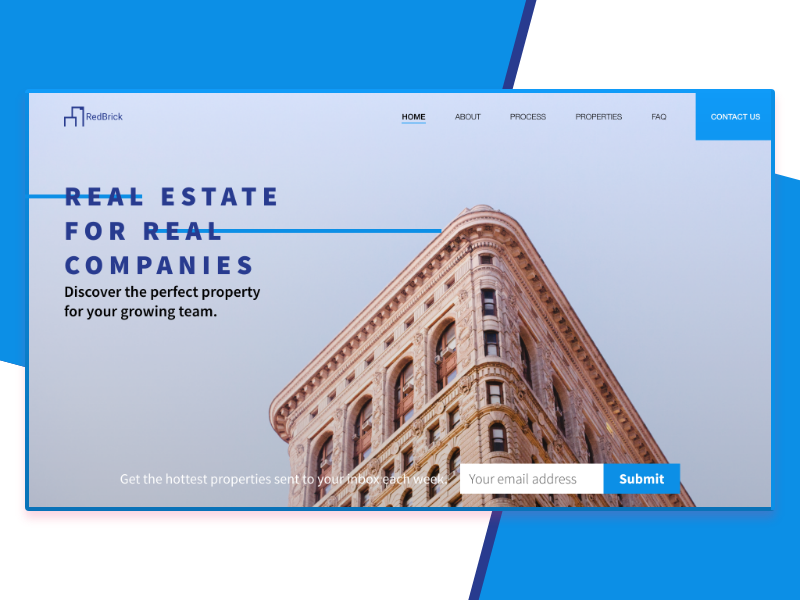The website's homepage for a real estate company features a sophisticated design with prominent red-brick elements at the top, flanked by two asymmetrical columns in a blue outline that suggests the façade of a classic building. The backdrop of the page is a sleek, modern gray, providing a sharp contrast to the vibrant blue elements.

On the right side of the page, starting from the center and extending to the right, is a neatly organized navigation menu including links to "Home," "About," "Process," "Properties," "FAQ," and "Contact Us." 

Towards the left side, the heading, "Real Estate for Real Companies," is displayed in bold blue text. The phrase "real companies" has a notable visual play, with a line striking through "real" and redirecting it towards the image of a stylish yet traditionally-designed building. This building features multiple windows and stories, embodying a blend of modern elegance and timeless architectural charm.

Underneath this heading, a call-to-action reads, "Get the hottest property sent to your inbox each week," accompanied by a field to enter your email address and a "Submit" button. The backdrop of this section is highlighted with abstract blue shapes on both the left and right sides, which then taper off towards the page's top and bottom edges, giving a balanced and aesthetically pleasing finish to the design.